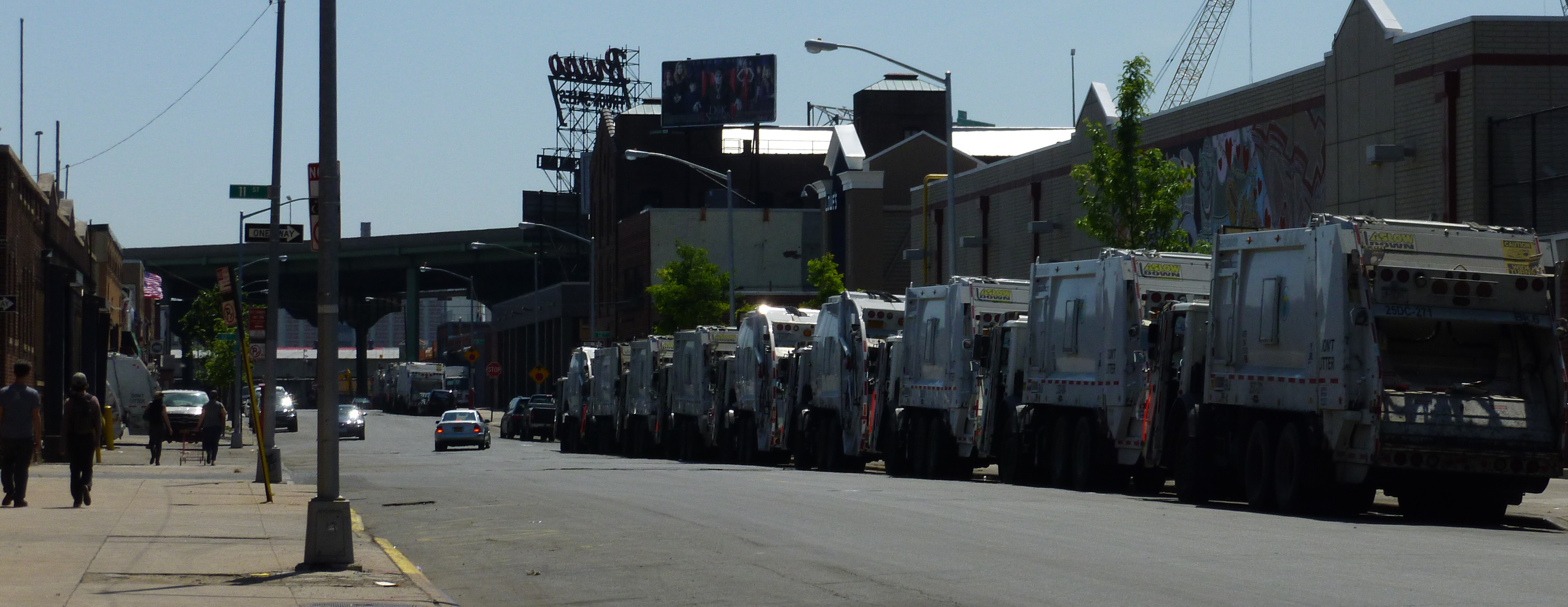The photograph captures a bustling city street on a bright day, with a notable line of nine white garbage trucks parked back to back along the right side of the road. Above the trucks, a large crane stretches skyward from behind tall buildings. The image also features a mixture of other street elements, including street lamps, billboards, and a stop sign. The left side of the picture showcases a yellow-painted curb and a sidewalk with four or five people walking, some with dogs. In the middle distance, a few cars can be seen driving on the road. Further down the street, there's a bridge crossing what appears to be a river. A bluish sky adds to the charm of the busy urban scene.